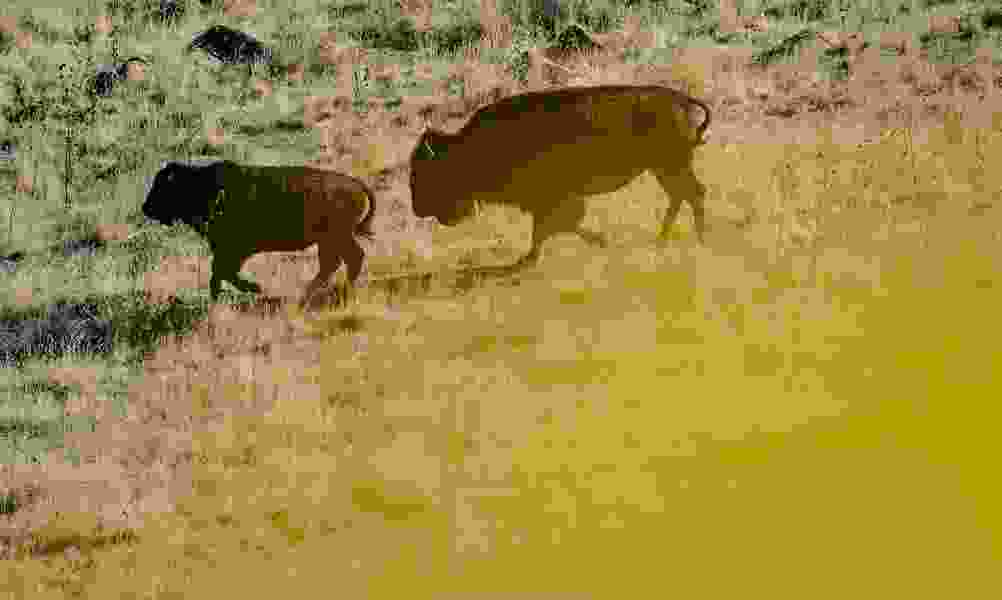The image depicts a field scene with two bison walking in profile from right to left across a grassy area scattered with patches of rocks. The central bison is larger and brown, while the smaller bison beside it, possibly its calf, appears dark near the head, and greenish-brown due to heavy pixelation. The background, particularly on the top left, shows light green grass interspersed with brown and black shapes, likely rocks. Unfortunately, the bottom right half of the image is heavily degraded with yellow and brown pixels, along with some lighter pink pixels, making the scene difficult to fully appreciate. The overall quality of the image is poor, with significant graininess and pixelation distorting the intended photorealistic style, rendering the finer details virtually indiscernible.